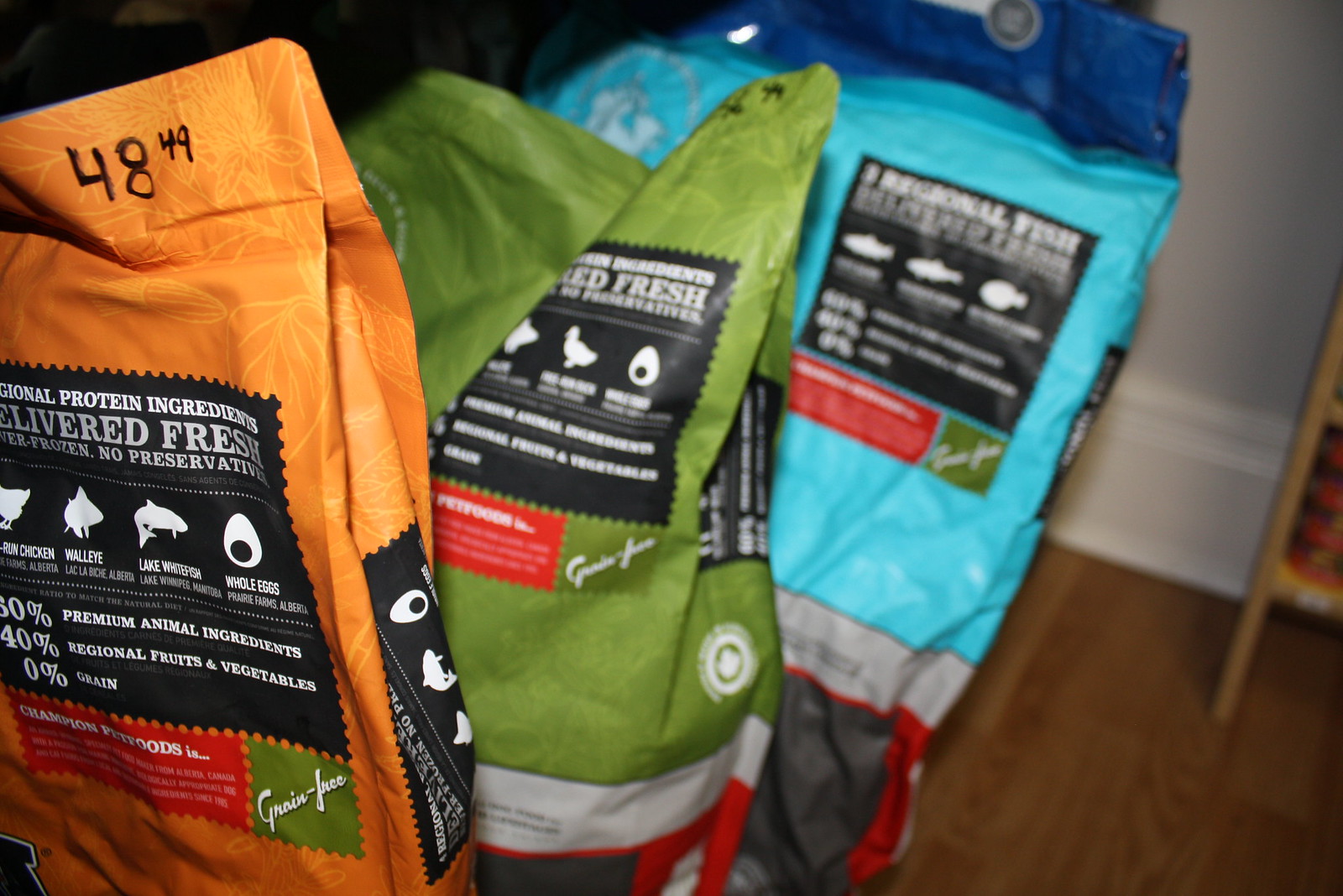The image depicts several colorful bags of pet food arranged on a brown wooden floor against a half-off-white wall with a white baseboard. The foreground features an orange bag with a black background and white lettering, stating "delivered fresh, no preservatives, protein ingredients." Illustrations of whole eggs, a lake fish, walleye, and the back half of a chicken are labeled accordingly, accompanied by text that reads "60% premium animal ingredients, 40% regional fruits and vegetables, 0% grain.” Below this is a red background with "Champion Pet Foods" written on it, along with a small green rectangle labeled "grain free" in white letters. Behind this is a teal-topped bag featuring shades of dark blue, light, and dark gray. The middle bag is olive green with similar black and red elements and white text saying "delivered fresh." All bags showcase illustrations of whole eggs, fish, and chicken, emphasizing the fresh regional protein ingredients they contain.